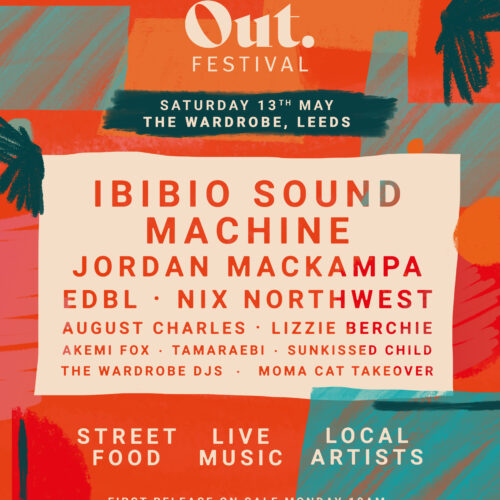This vibrant advertisement for an upcoming festival radiates with a burst of orange and red hues, complemented by subtle teal square and rectangle shapes, giving it a faintly painted aesthetic. The event is named "Out. Festival" and proudly showcases its details at the top: "Saturday, 13th May, The Wardrobe, Leeds," with "Leeds" boldly spelled out. The advertisement lists an impressive lineup of performers including Ibibio Sound Machine, Jordan Mackampa, EDBL, Nicks Northwest, August Charles, Lizzie Berchie, Akey Fox, Tambora, Sun-Kissed Child, The Wardrobe DJs, and Mama Cat Takeover. Adding to the tropical vibe, there are hints of palm trees in the background. Most of the text is presented in a beige color, harmoniously tying in with a beige rectangle that stands out in the center. Emphasizing the festival's offerings, the bottom of the ad highlights in beige letters: "Street Food, Live Music, and Local Artists." This visual delight is not just an invitation, but a promise of an unforgettable experience filled with culinary delights, rhythmic tunes, and artistic flair.